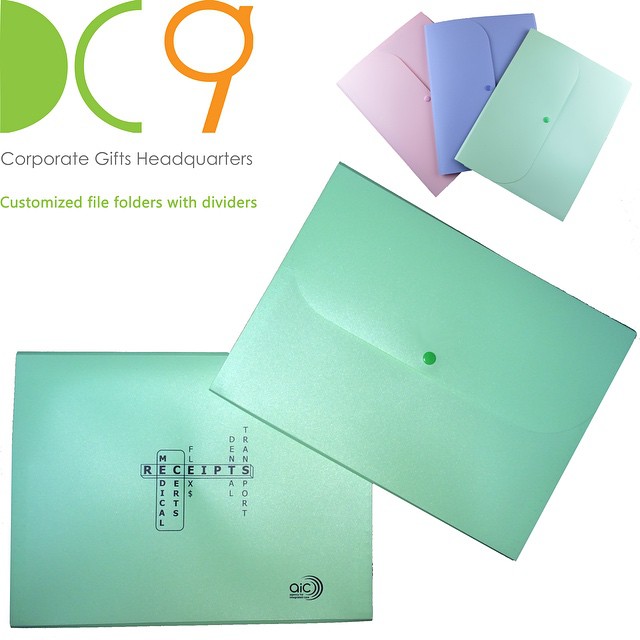This image depicts an advertisement for file folders from a brand possibly identified as DC9 or DCG, featuring a stylized green and orange logo. The top left corner displays the text "Corporate Gifts Headquarters," followed by "Customized File Folders with Dividers" in green. The background is a uniform white, emphasizing the product details.

In the upper right of the image, there are three pastel-colored folders arranged from left to right in purple, mint, and pink. At the bottom of the advertisement, a larger image showcases a light green folder. The front side of this folder has a crossword-like pattern with the words "Receipts" horizontally, and "Medical Certs, Flex Dollars, Dental, and Transport" branching out vertically. The folders feature a unique flap mechanism secured by a green button, suggesting they are designed for organizing medical certificates and receipts, possibly hinting at use in a medical office.